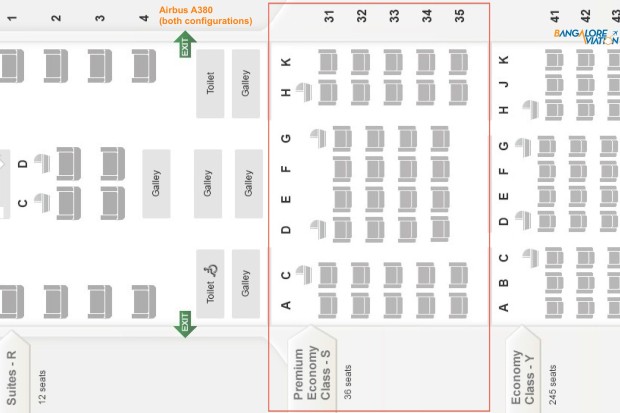This image displays a sideways view of an airplane seating map for Bangalore Aviation, specifically for the Airbus A380 in both configurations. The map is divided into three distinct sections, each with detailed annotations.

On the left side, marked in yellow, are the accommodations for First Class, featuring 12 spacious suites. Important amenities such as exits, toilets, and galleys are clearly labeled, highlighting the luxurious and roomy layout of this section.

The middle section, outlined with a red line to indicate it is currently selected, showcases rows 31 to 35 in the Premium Economy Class. This area has 36 seats arranged in a 2-4-2 configuration, offering more space compared to Economy Class.

The rightmost section details the Economy Class, covering seat rows from 41 onwards. With a total of 245 seats laid out in a 3-4-3 formation, this section is more densely packed, reflecting the limited personal space typically found in standard economy seating.

Overall, the map illustrates the seating arrangements across different classes, emphasizing the varying levels of comfort provided by First Class, Premium Economy, and Economy Class.